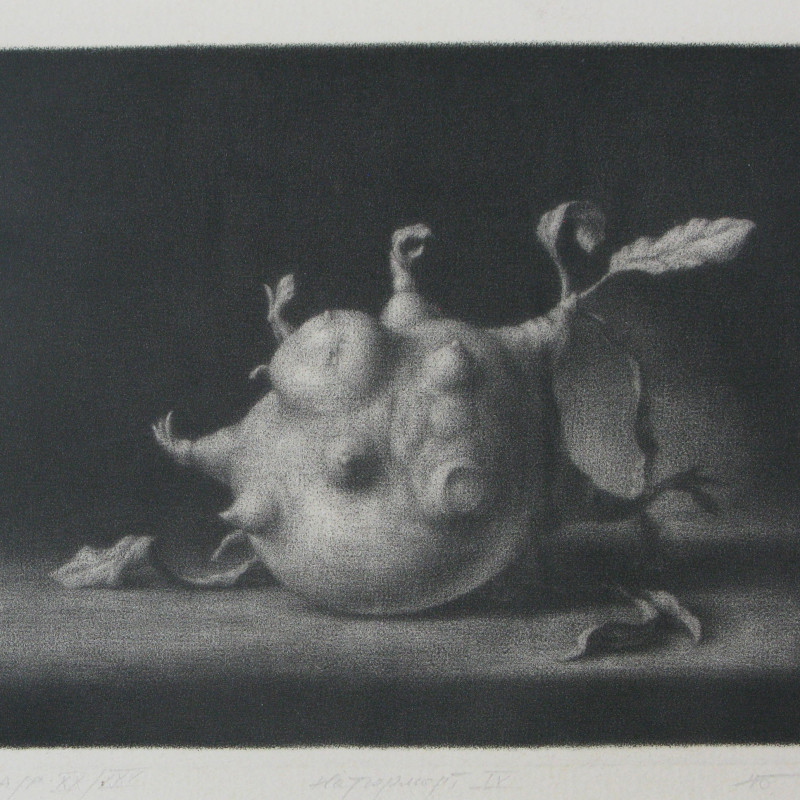The image depicts a black and white painting featuring a large, round, and lumpy root vegetable, resembling a potato or turnip. The vegetable is characterized by numerous bumps and wiry sprouting structures across its surface, with some sprouts resembling human hands or nipples. It has multiple root-like extensions; notable ones include a large bump at the top left, horn-like structures on the right, and several around the base. Leaves are emerging from various parts, particularly the top right and the bottom. The background is predominantly dark, with varying shades of black and charcoal gray, creating a heavily shaded atmosphere. Additionally, the image includes a distinctive long white strip at both the top and bottom, and the ground features a mix of black and white colors, adding to the intricate details of the scene.